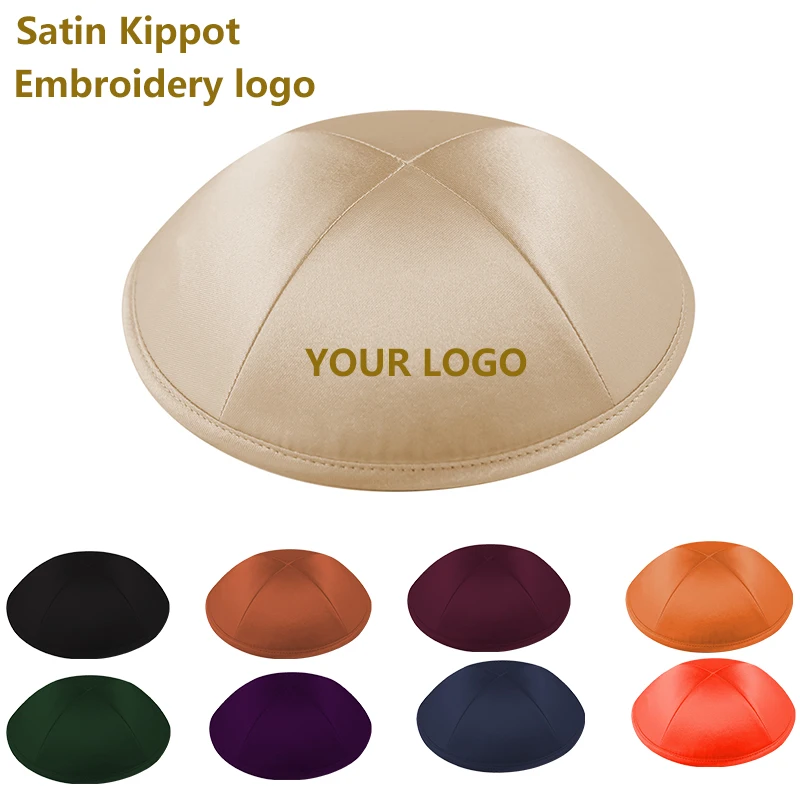This is a detailed, color photograph serving as an advertisement for satin kipot, traditionally known as yarmulkes, featuring customizable embroidered logos. At the top left corner of the advertisement, golden text reads "Satin Kipot Embroidery Logo." Centrally displayed is a large, tan-colored satin kipah bearing the placeholder text "Your Logo" in gold, signifying the customizable nature of the product. Below this central example, the advertisement features eight smaller kipot in an array of colors including black, green, bronze, purple, wine, dark blue, red, and gold. The entire display is set against a white background, emphasizing the richness and variety of available hues. This photograph effectively showcases the versatility of the kipot, inviting potential buyers to envision their own logos embroidered on these elegant, brimless caps that fit snugly atop the head.